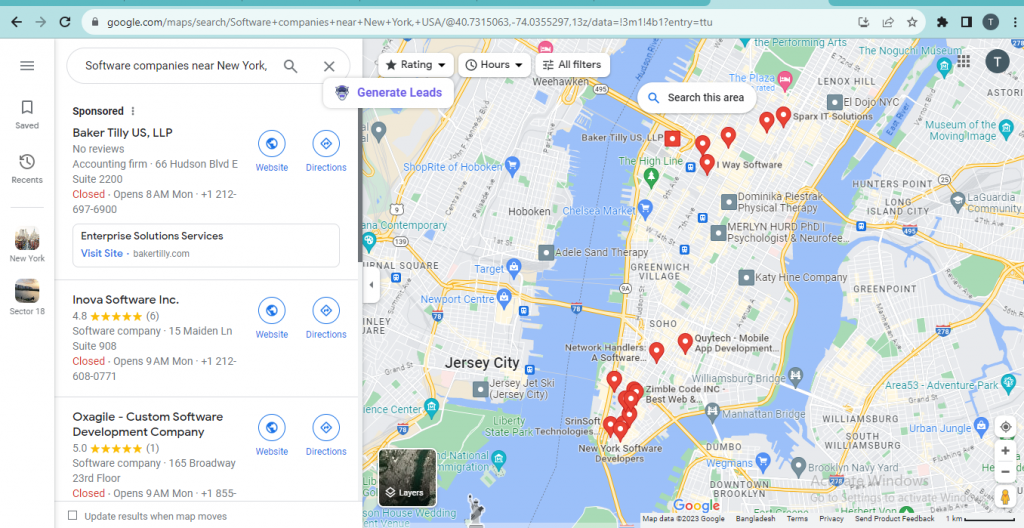The image depicts a screenshot of Google Maps as viewed on a web browser. The browser interface is visible, including elements like the web address bar situated at the upper center of the image, along with navigation buttons such as the back arrow, forward arrow, and refresh button. 

On the left-hand side, there is a vertical menu comprising five items. The first item shows three horizontal bars, which usually indicate a menu icon. Below this are sequentially listed items labeled "Saved" and "Recents." 

Further down the menu, a gray separator demarcates a new section featuring location labels "New York" and "Sector 18." To the right of this section, another vertical menu lists three business entries. The first business is a sponsored listing for "Baker Tilley's US LLP." Following this is "Innova Software Incorporated" and "OXAGILE Custom Software Development Company." 

This combination of elements provides a detailed visual breakdown of the Google Maps interface as captured within a web browser.